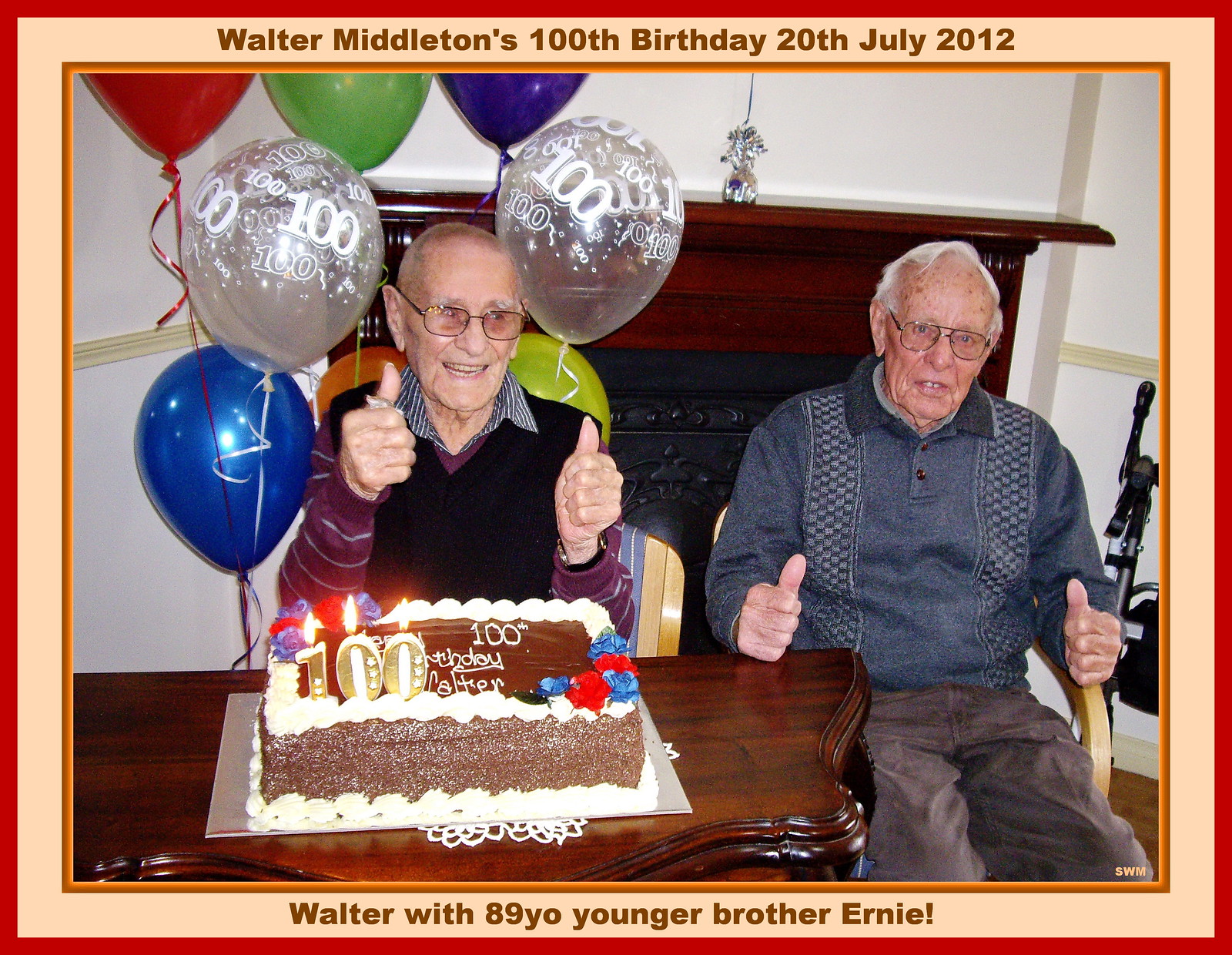This is a framed photograph commemorating Walter Middleton's 100th birthday on July 20th, 2012. The red, tan, and orange border at the top reads, "Walter Middleton's 100th birthday, 20th July 2012," while the bottom caption states, "Walter with his 89-year-old younger brother, Ernie." 

Seated on the left side of the image is Walter Middleton, who joyfully has both thumbs up. Walter is wearing glasses, a black sweater vest over a purple shirt with a collar, and he appears notably content. Positioned behind him are white balloons emblazoned with the number 100, and a blue balloon to his left. In front of him sits a chocolate cake with white icing, bearing the message "Happy 100th Birthday, Walter" and topped with three lit candles forming the number 100.

To Walter's right is his younger brother, Ernie, who also has both thumbs up. Ernie sports glasses, a navy blue shirt, and dark pants. Unlike Walter, Ernie has a head of light white hair. The brothers are captured in a moment of shared celebration, surrounded by the festive ambiance of balloons and the joy of reaching a remarkable milestone together.

The photograph, which is placed on a beautifully wooden antique table, radiates the warmth and happiness of the occasion, encapsulating the jovial spirit of Walter's centennial celebration alongside his beloved younger brother.